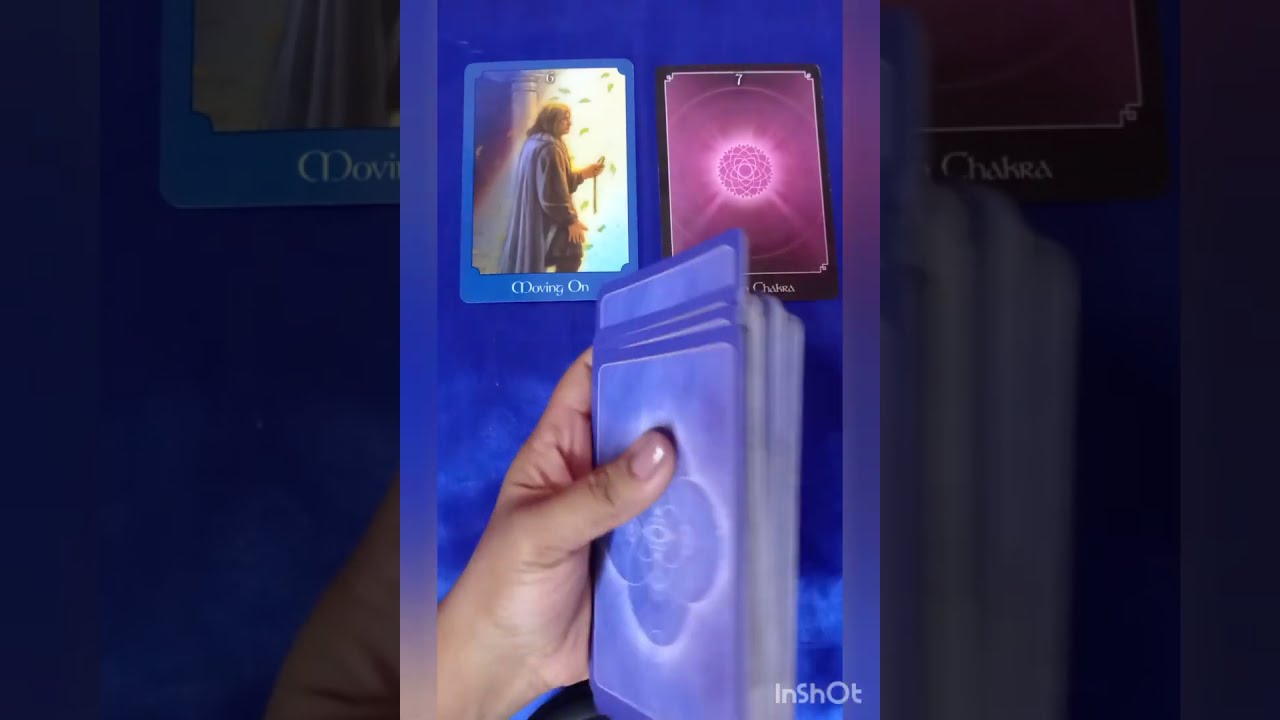The image depicts a photograph with a hand, likely brown-skinned, holding a deck of tarot cards against a blue background with a cloudy appearance. The purple cards have a floral or geometric pattern in the center. In the foreground, two cards are prominently displayed. The first card shows a person in a long robe, walking from a dark interior into a bright outdoors with falling leaves, labeled "Moving On." The second card features a luminous purple mandala with a black border and the word "chakra" written underneath. The photo is marked with the "InShot" logo in white text at the bottom right corner, indicating it could be a screenshot from a video edited using the InShot app. The overall image has a slightly darker, blurred background, making the central elements stand out more vividly.